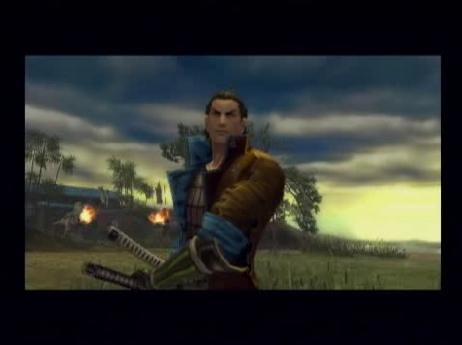In this screenshot from a video game, a male character is prominently featured. He is wearing a distinctive leather jacket, which has a striking blue lining on the inside. The jacket is adorned with various details and accessories, contributing to his rugged appearance. The character's left hand rests confidently on the hilt of his swords, suggesting readiness for combat. His stance and attire indicate a seasoned warrior or adventurer, poised for action in the immersive world of the game.